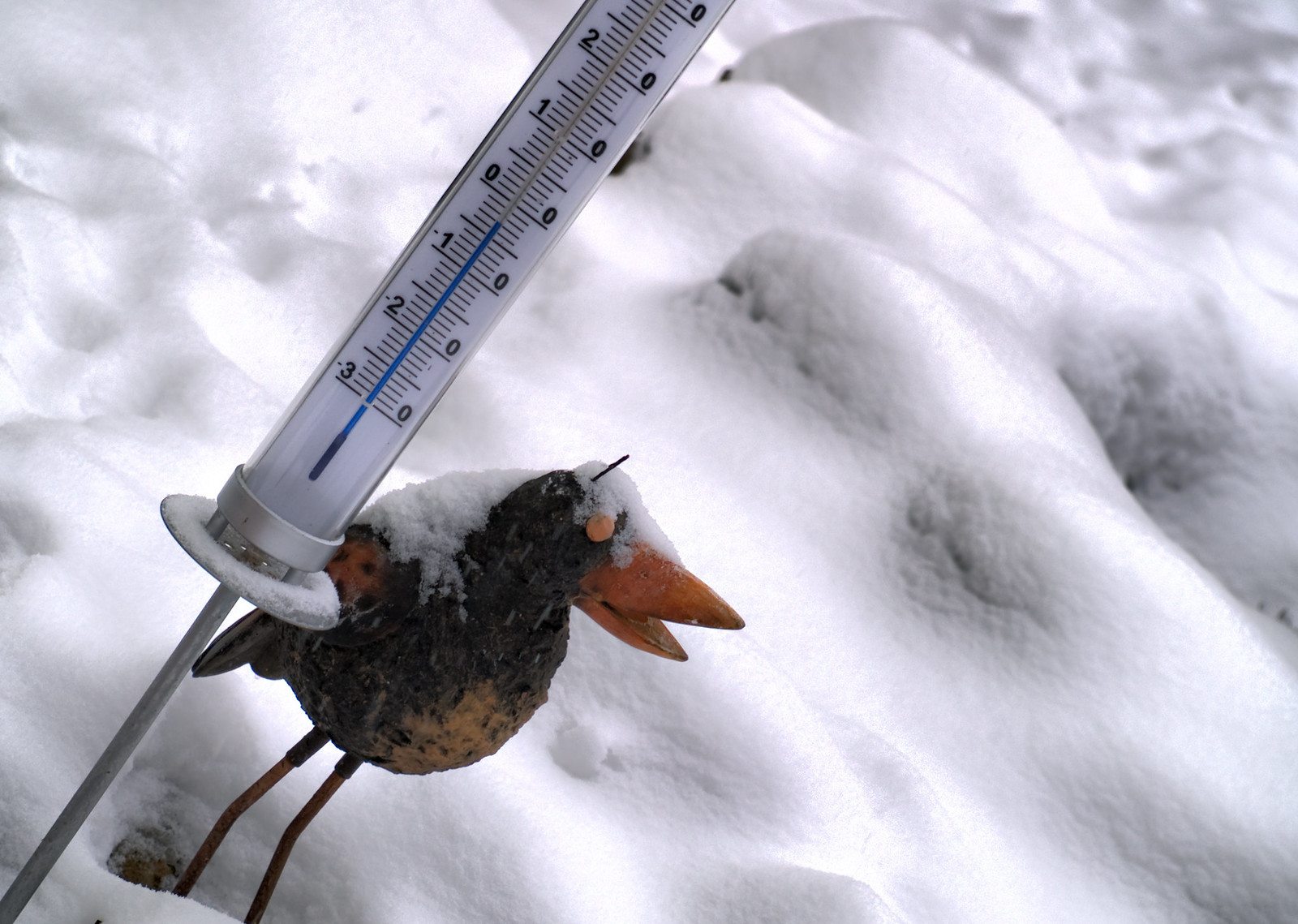A high-resolution outdoor photograph taken on a sunny, snow-covered day featuring a close-up view of a thermometer positioned in the ground. The thermometer showcases a sleek design with a long, silver metallic stake at its base, firmly embedded in the snow. The thermometer's glass tube displays mercury colored in a striking blue hue, indicating a near-freezing temperature of approximately -0.5 degrees. The calibrated scale consists of black numerals on a pristine white background, ranging from -3 to 2 degrees, with the zero mark prominently displayed on the opposite side of the mercury column. Adjacent to the thermometer, a meticulously sculpted, long-legged bird with an orange beak stands as a charming decorative element, its back blanketed in a thick layer of pristine snow. The entire scene is enveloped in glistening snow, emphasizing the serene and chilly atmosphere of the winter day.